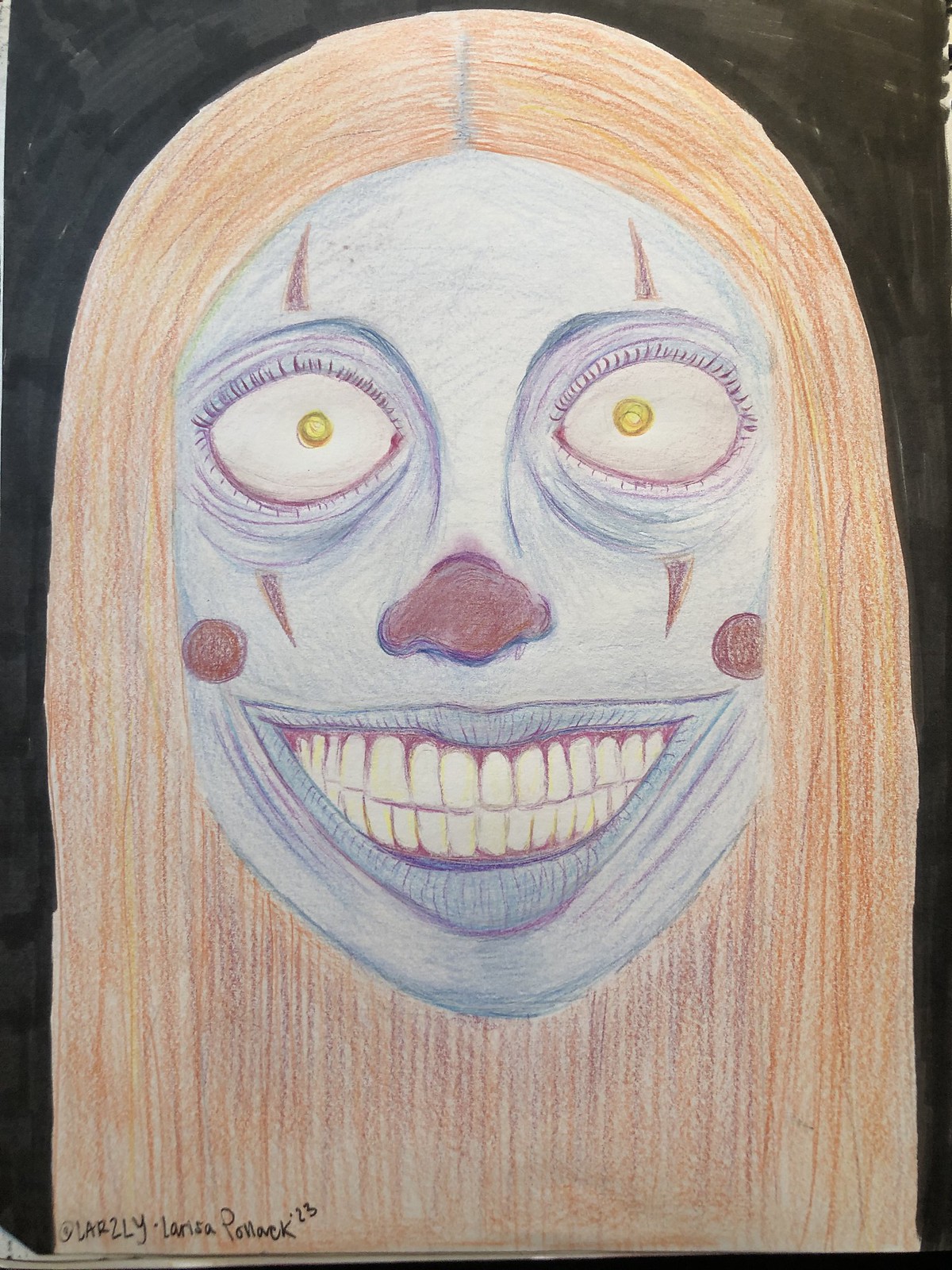The illustration depicts a sinister clown with a floating, disembodied head set against a stark black background. Created using crayons or colored pencils, the ominous figure stares directly into the viewer's eyes with an unsettling intensity. Its face bears a bluish-gray hue, adorned with a wide, crooked grin that exposes long, white teeth, and accentuated by wrinkles around the mouth. The clown's thin lips are purple, and its gums are slightly visible above and below the teeth.

Its eyes are wide and circular, completely white except for yellow pupils at the center. Encircling the eyes are red rims with short lashes and further emphasized by elongated, horn-shaped red streaks both above and below. The nose is small yet vividly red at the tip, in classic clown fashion.

Additional facial features include two red circles on each cheek, suggesting blush, contributing to the overall menacing appearance. The hair, parted down the middle, extends in dark blonde strands all the way to the bottom of the page. The artist's signature, rendered in black pencil or ink, is situated at the bottom left of the image, completing this eerie visual.